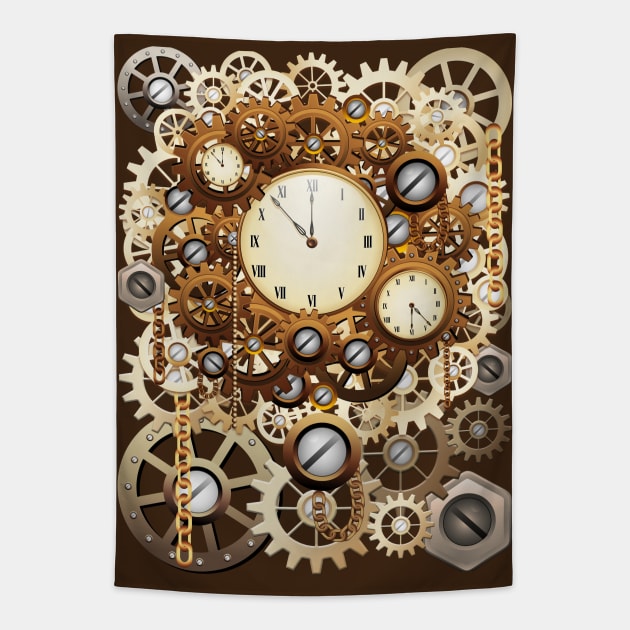The image showcases a meticulously detailed, computer-generated tapestry featuring an intricate assemblage of gears and clocks. Central to the image is a large clock with Roman numerals, displaying the time at 11:53, its shorthand on the 12 and longhand just before the 11. Flanking this main clock are two smaller clocks set diagonally, one positioned at the top left and the other at the bottom right, both showing the same time, though the bottom right clock is slightly larger and depicted upside-down. The entire tapestry is adorned with a variety of copper-colored gears of different sizes, all interlinked and aligned, creating a harmonious network of mechanisms that suggest perpetual motion. Scattered throughout the scene are additional elements like dangling gold chains and slots for slotted screwdrivers, adding to the intricate and somewhat enigmatic beauty of the design.